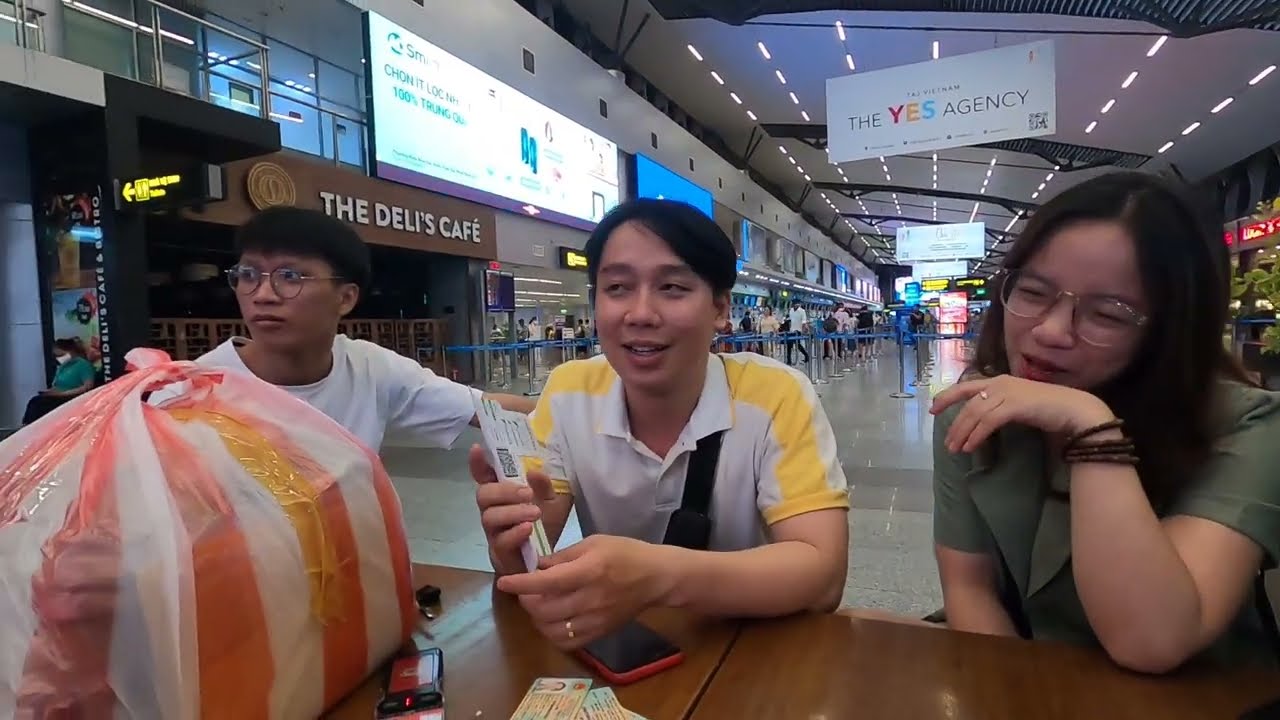The photo captures three Asian teenagers, likely high school students, seated at a table within a shopping mall. From left to right, the first individual is a male with short black hair and round glasses, wearing a white t-shirt, and looking off to the left. The middle individual, also a male with short black hair, wears a white and yellow polo shirt and is holding what appear to be airline tickets or possibly IDs in his hand, while also looking to the left. The third person on the right is an Asian girl with long black hair and round glasses, wearing an olive green short-sleeved top; she has her eyes closed and is looking downward, possibly at the table. On the table in front of them, which is of medium dark wood, lies a collection of items, including IDs, a red phone, and a key. In the foreground to the bottom left is an orange and white striped bag, knotted at the top. The backdrop features a variety of mall stores, including 'Deli's Cafe' and 'The Yes Agency,' indicating a bustling shopping environment.